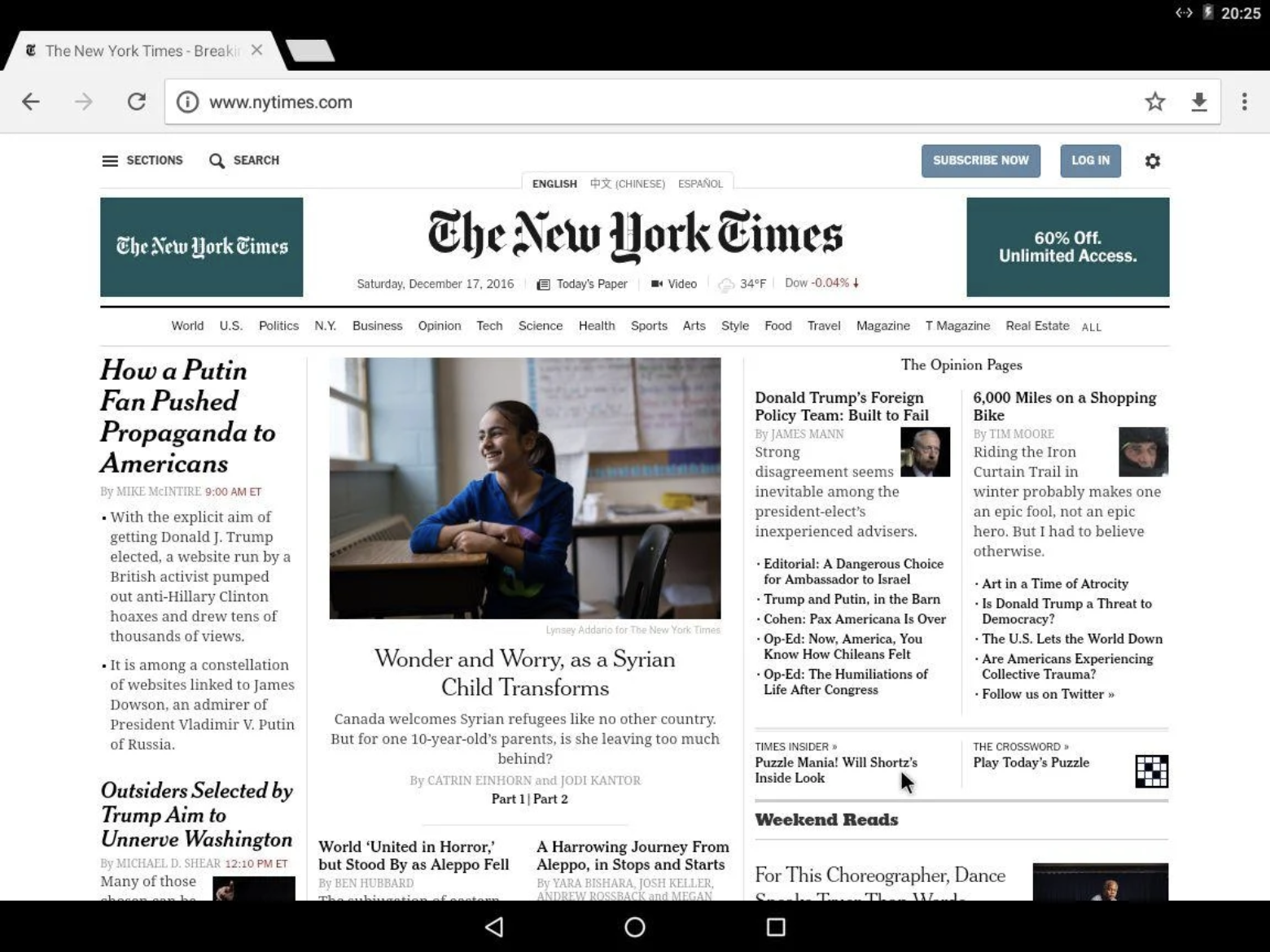A New York Times webpage is open, displaying the various sections available for reading including 'World,' 'U.S.,' 'Politics,' 'New York,' 'Business,' 'Opinion,' 'Tech,' 'Science,' 'Health,' 'Sports,' 'Art,' 'Style,' 'Food,' 'Travel,' 'Magazine,' 'T Magazine,' and 'Real Estate.' The headline "How Putin Fan Pushed Propaganda to Americans" is prominently featured, discussing a British-run website's efforts to disseminate anti-Hillary Clinton content with the goal of electing Donald J. Trump. Other featured headlines include "Outsider Selected by Trump Aims to Unnerve Washington," "World United in Horror but Stood By as Aleppo Fell," and "A Harrowing Journey from Aleppo in Stops and Starts." The opinion section highlights an article titled "Donald Trump’s Foreign Policy Team Built to Fail," amidst other varied content. The webpage dates back to Saturday, December 17, 2016, showcasing a mix of political, global, and social issues.